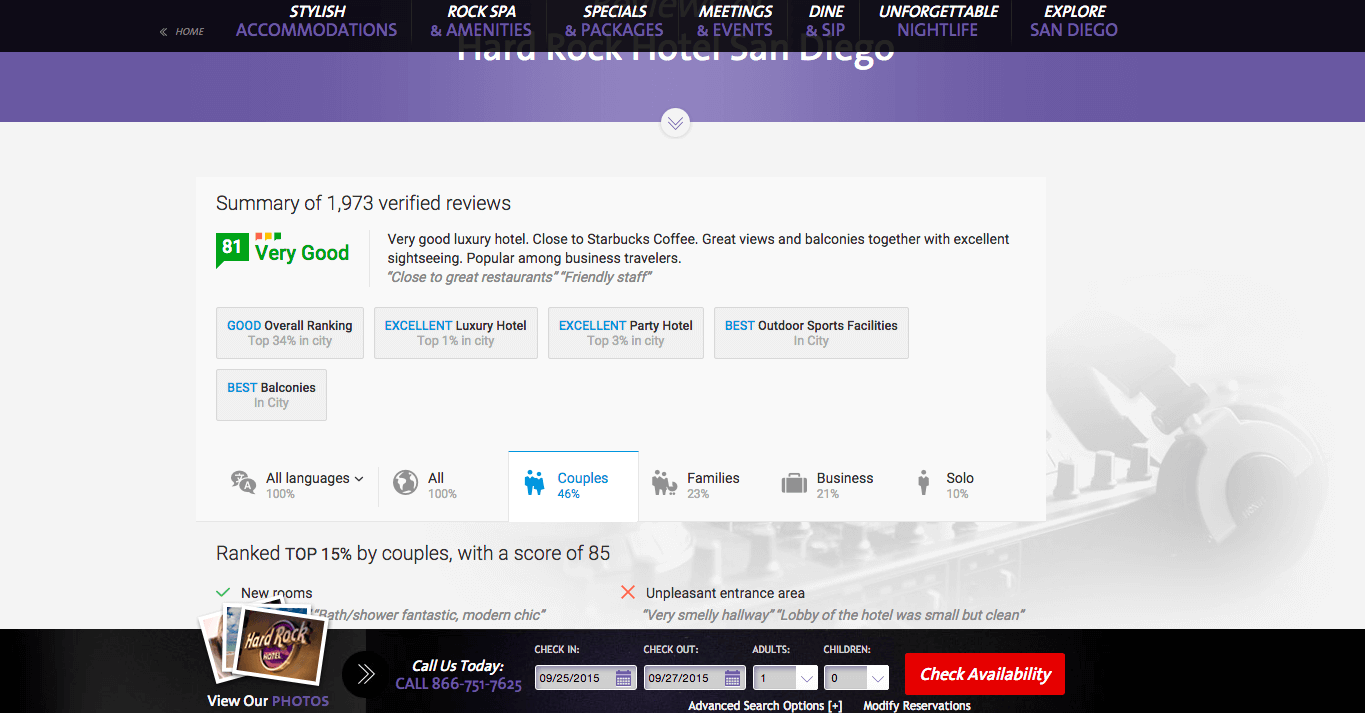The image showcases a webpage or application interface for the Hard Rock Hotel in San Diego. At the top, there's a sleek black navigation bar featuring clickable options: "Home," "Stylish Accommodations," "Rock Spa and Amenities," "Specials and Packages," "Meetings and Events," "Dine and Sip," "Unforgettable Nightlife," and "Explore San Diego." Each section header is styled consistently with "Stylish" in white and the subsequent word in purple.

The partial top banner confirms the hotel name, "Hard Rock Hotel San Diego," though partly obscured by the black bar. Scrolling down reveals detailed highlights and reviews. The homepage summary includes information from 1,973 verified reviews, with an overall rating of 81, labeled as "very good." Specific feedback points out the hotel's proximity to Starbucks, excellent views, balconies, and prime sightseeing opportunities, making it popular among business travelers. Additionally, it praises the friendly staff and nearby great restaurants.

The interface also displays accolade sections, such as the hotel being rated as a "Very Good Luxury Hotel," having the "Best Outdoor Sports Facilities," the "Best Balconies," and being an "Excellent Party Hotel." Guest segmentation data at the bottom shows the types of visitors: 46% couples, 23% families, 21% business travelers, and 10% solo travelers.